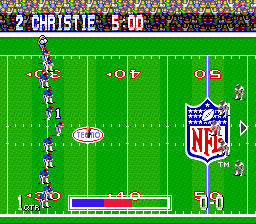This image appears to be a still from a vintage video game with dated graphics, showcasing a classic football scene. The setting is a verdant green field marked with white yard lines at intervals, including the numbers 50, 40, and 30, progressing from right to left. Centrally located on the field is the iconic NFL logo in red. 

Clustered along the yard line near the 30-yard marker is an assembly of football players donned in blue and white uniforms, poised for action. In the lower part of the image, a colored status bar is visible; it transitions from blue on the left, through a red middle section, to green on the right, with the numbers '00' displayed in the right corner.

At the bottom of the image, a scoreboard or status bar is visible, with a gradient transitioning from blue on the left, red in the center, and green on the right, with '00' in the right corner. 

Additionally, two football players in white and black uniforms stand over the NFL logo. Text in the upper left corner, possibly floating over a rendered crowd, reads "2 Christy 5 o'clock."

This meticulously captured scene not only evokes nostalgia but also highlights the simplicity and charm of early sports video games.